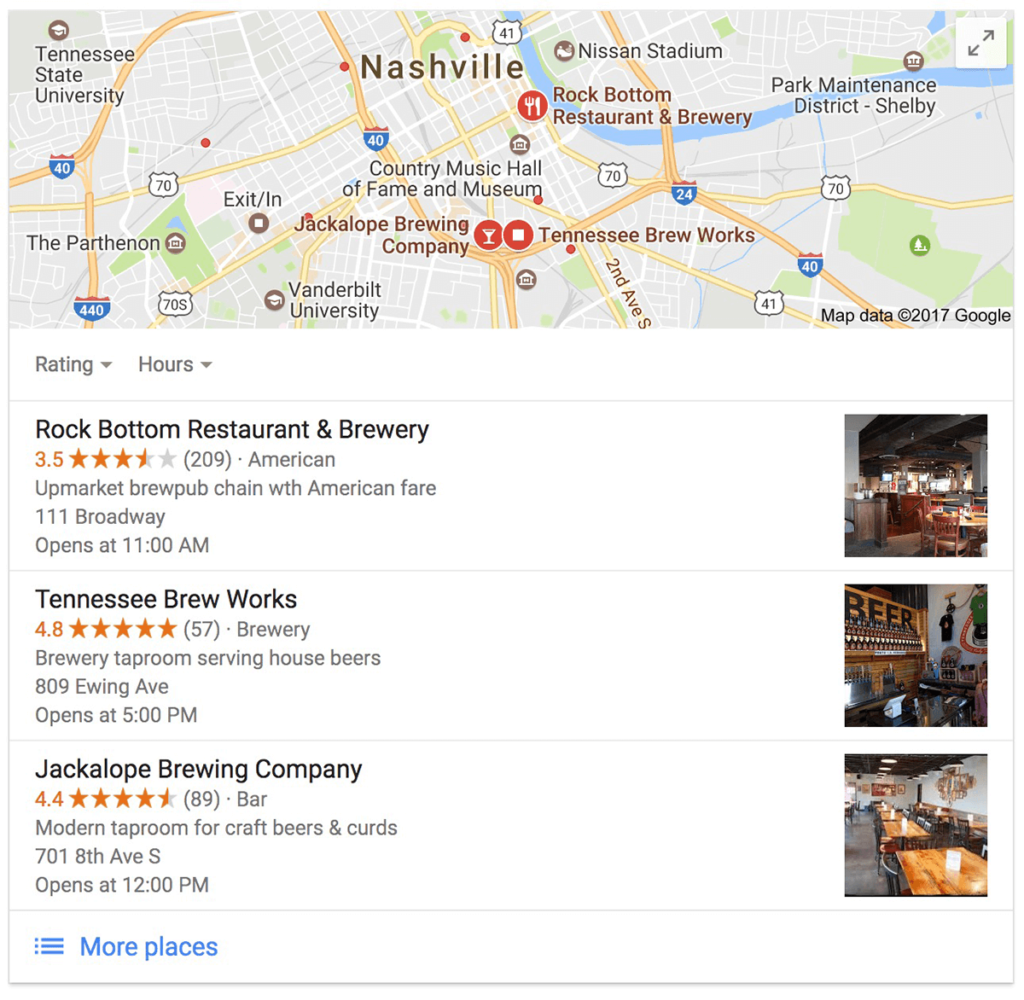The screenshot captures a detailed Google search results page highlighting popular breweries in Nashville, Tennessee. At the top of the screen, there is a map of Nashville, featuring notable landmarks such as the Country Music Hall of Fame, Vanderbilt University, and The Parthenon, alongside the city's intricate street layout.

Prominently marked on the map are three featured breweries:

1. **Rock Bottom Restaurant and Brewery**:
   - **Address**: 111 Broadway
   - **Type**: Upmarket brew pub chain serving American fare
   - **Opening Hours**: 11 a.m.
   - **Rating**: 3.5 stars from 209 reviews

2. **Tennessee Brew Works**:
   - **Address**: 809 Ewing Avenue
   - **Type**: Brewery taproom serving house beers
   - **Opening Hours**: 5 p.m.
   - **Rating**: 4.8 stars from 57 reviews

3. **Jackalope Brewing Company**:
   - **Address**: 701 8th Avenue South
   - **Type**: Modern taproom offering craft beers and curds
   - **Opening Hours**: 12 p.m.

Below the map, the search results are listed in detail, consistent with the markers above. Additionally, the page includes options to explore more places via a clickable button, and an option to enlarge the map for a better view. This concise search result provides a snapshot of key brewery options for those exploring Nashville's vibrant beer scene.